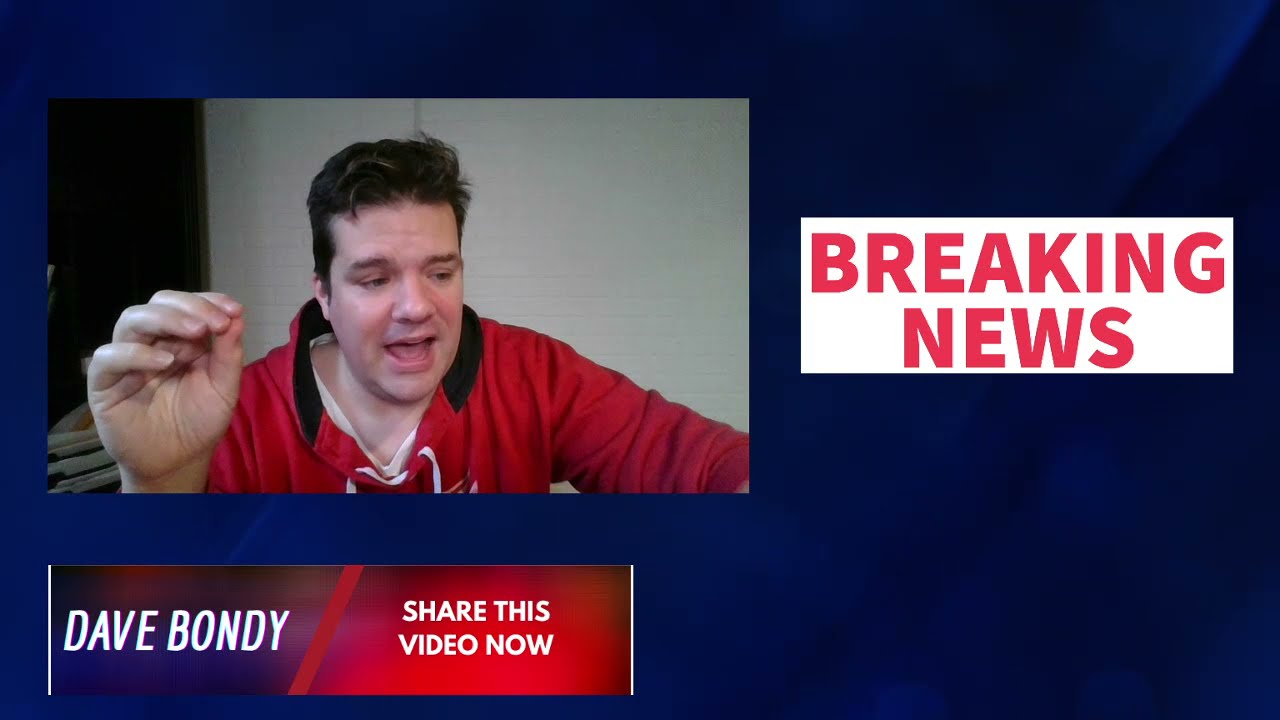In this live stream screenshot, the image features a white-skinned man, identified as Dave Bondy, set against a dark blue background. The man, positioned on the left half of the image, appears to be speaking authoritatively, wearing a red hoodie and displaying a gesture with his right hand, where his forefinger and thumb are pinched together. He seems to be in a domestic setting, likely a lounge or bedroom, possibly with a few books behind him. Prominently displayed in massive red capital letters to the right of the image is the announcement "Breaking News," emphasizing the urgency of the message. Below the man’s image, there is a blue and red banner with the text "Dave Bondy" and an imperative call to action, "Share this video now," indicating this could be a live stream from a YouTube video or another platform where breaking news is being discussed. The overall layout and color scheme suggest a formal presentation style, akin to a PowerPoint slide.